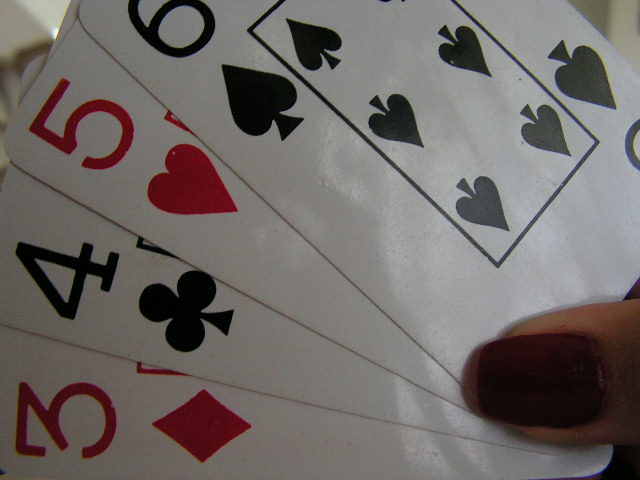This is a horizontally-oriented, close-up photograph capturing a detailed view of a hand holding a fan of playing cards. The thumb, adorned with a long nail polished in a deep, dark blood-red color, is prominently visible in the bottom right corner. The topmost card in the fan is the Six of Spades, showcasing black spades on a white background. Partially visible beneath the Six of Spades is a Five of Hearts, displaying red hearts. Following this, you can see the edge of the Four of Clubs, with its black clubs. Finally, the Three of Diamonds, with red diamonds, is just barely visible at the bottom. The alignment and orientation of the cards create a layered effect, offering a clear view of the Six of Spades while hinting at the sequence of cards beneath it.